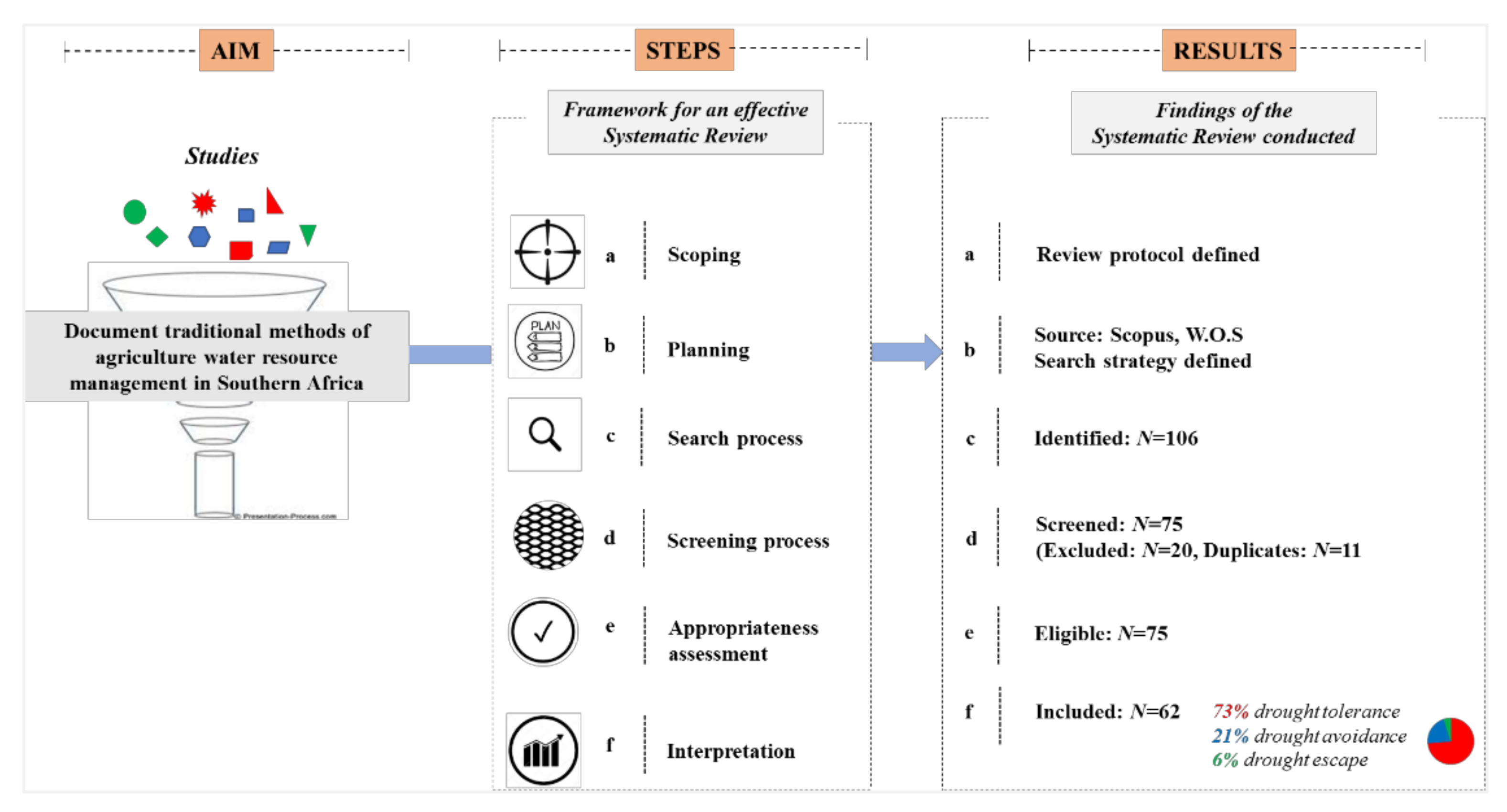The image depicts a scientific chart with three distinct columns labeled "AIM," "STEPS," and "RESULTS," presented against a white background. The "AIM" column includes a detailed description of documenting traditional methods of agriculture and water resource management in Southern Africa, illustrated by various geometric shapes—circles, squares, and other colored shapes (green, blue, and red)—appearing to be funneled through a chalice-like diagram. The "STEPS" column outlines the framework for an effective systematic review, starting from "Scoping" to "Planning," followed by "Search Process," "Screening Process," "Appropriateness Assessment," and "Interpretation," each represented by specific icons such as magnifying glasses and checkmarks, organized in a sequential manner (A to F). Lastly, the "RESULTS" column provides a detailed breakdown of the systematic review process, including statistics such as the number of sources identified (N=106), screened (N=75), excluded (N=20), duplicates (N=11), eligible (N=75), and included (N=62). It concludes with a pie chart illustrating the distribution of findings: 73% drought tolerance, 21% drought avoidance, and 6% drought escape, using green, blue, and red segments.